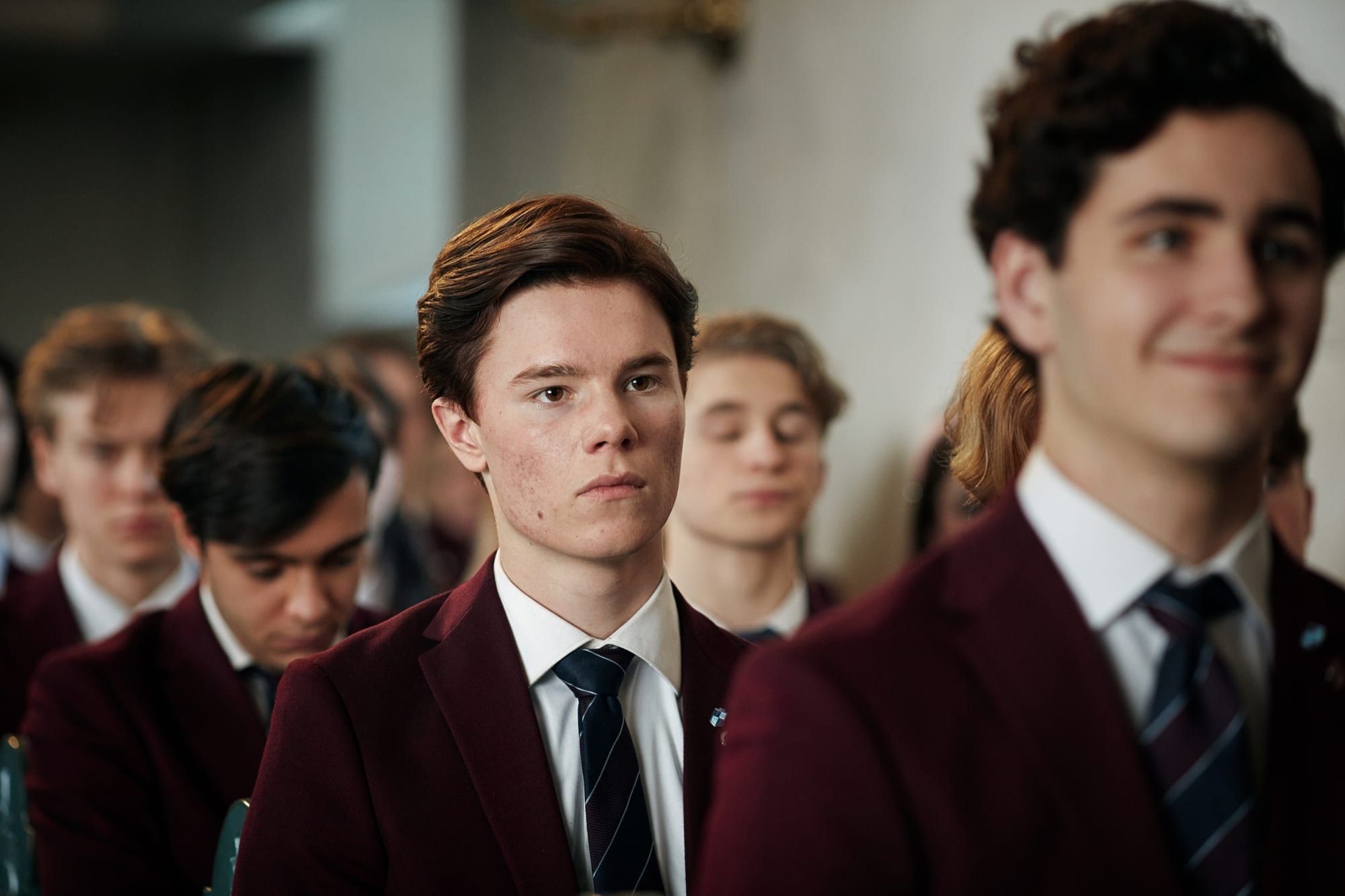The image showcases a group of teenage boys, approximately 15-16 years old, posed in their school uniforms, which consist of burgundy sports jackets, white collared shirts, and navy blue ties with diagonal burgundy and white stripes. At the forefront of the picture, there is a boy with curly, short black hair, smiling, though he appears slightly out of focus. Directly behind him stands another boy, the main focus, who has slightly reddish-brown hair brushed back, and an expression that can be described as a mix of sadness and contemplation. To his side, there is another boy with brownish-black hair looking downward. Further behind these three, additional boys are lined up, their features blurred but distinctively wearing the same uniform. The background is a grey wall, casting some shadows. The composition suggests a formal school setting, possibly a boys' school, with everyone dressed uniformly and the atmosphere muted in tone.